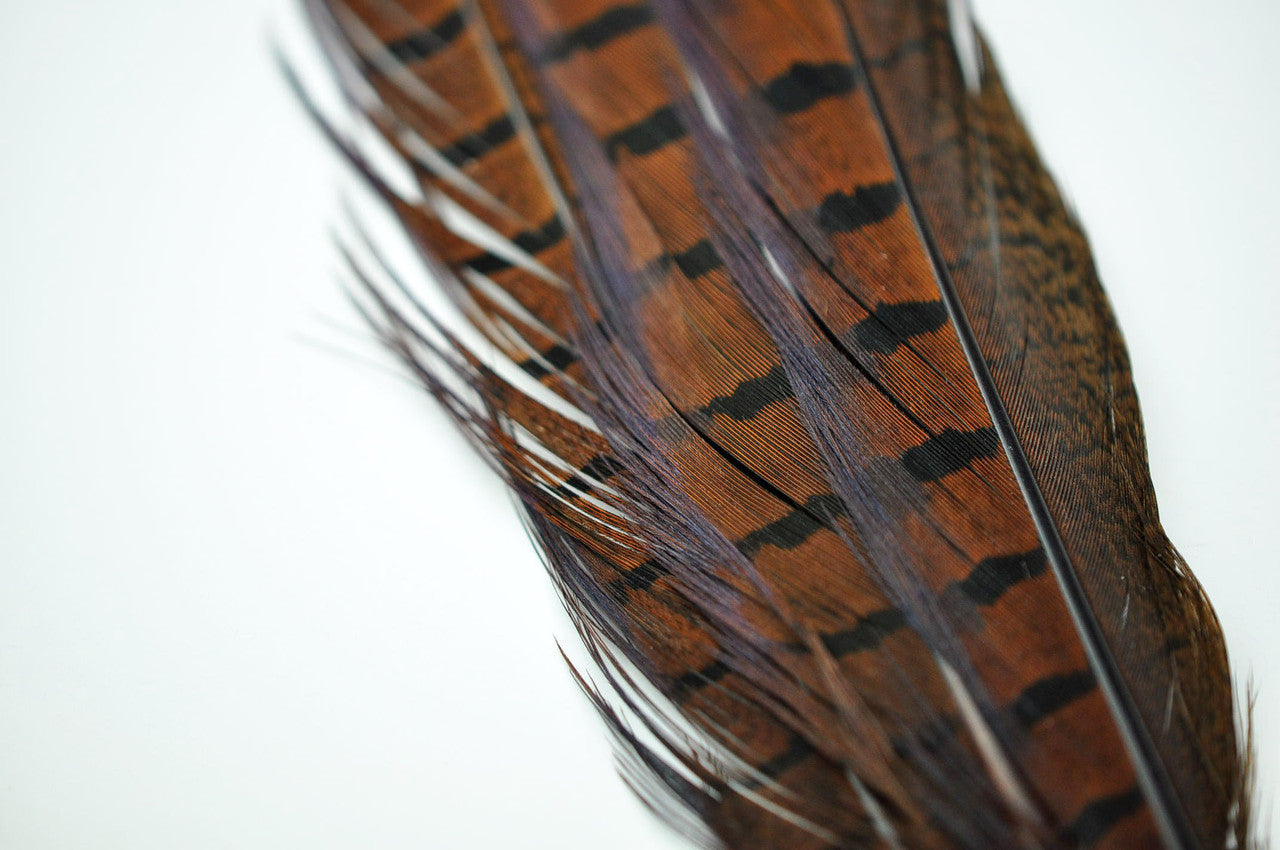This is a rectangular photograph, approximately six inches wide by three inches high, featuring a very close-up view of potentially two or three overlapping feathers. The background is a plain light blue-gray, almost white. Dominating the image, from the lower right-hand side extending towards the top center, is a large brown feather. The feather starts at about an inch and a half wide at the base and flares out to roughly two inches towards the top. 

The feather's central shaft is marked by a distinct, thin black line. On the right side of the shaft, the feather is a dark mahogany brown peppered with small black specks. On the left side, there are thick bands of reddish-brown interspersed with smaller horizontal bands of black. One side of the feather shows signs of separation with little slits, possibly from wind, adding a textured, silky-soft appearance that seems almost touchable. The intricate detail captures each individual grain, enhancing the sense of realism.